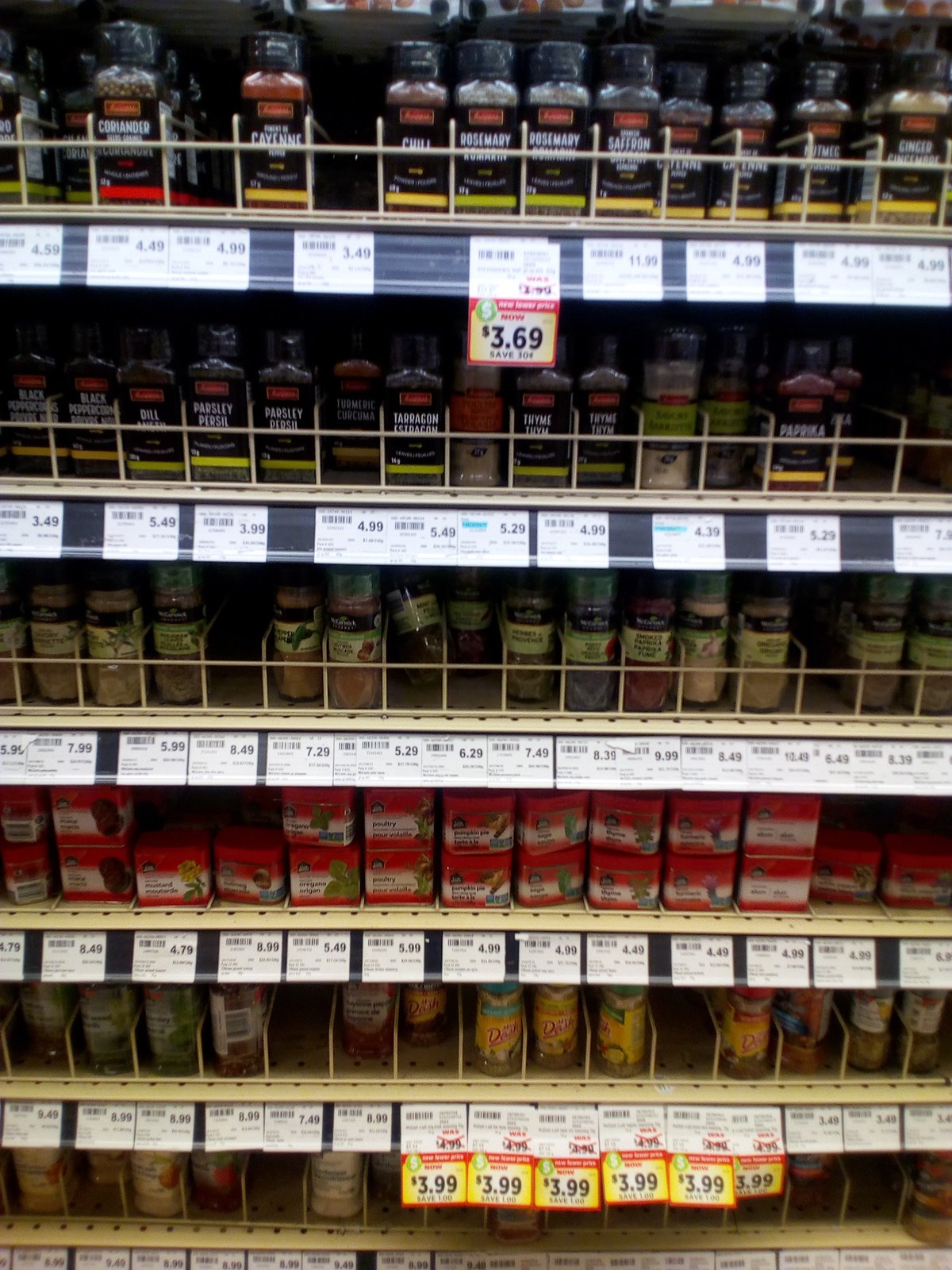The image captures a section of supermarket shelves, specifically five visible rows displaying various products. There are a total of six shelves, although the bottom shelf is only partially visible. Each product is marked with a white label, some adorned with yellow stickers, likely indicating discounted prices. Bottled goods dominate the shelves, with a notable exception in the center where a row of red boxes, possibly containing juice or tea, stands out. Blue and white labels on the upper shelves seem strategically placed to attract shopper attention. The overall scene conveys a well-organized retail display, with clear efforts to highlight special offers and key products.